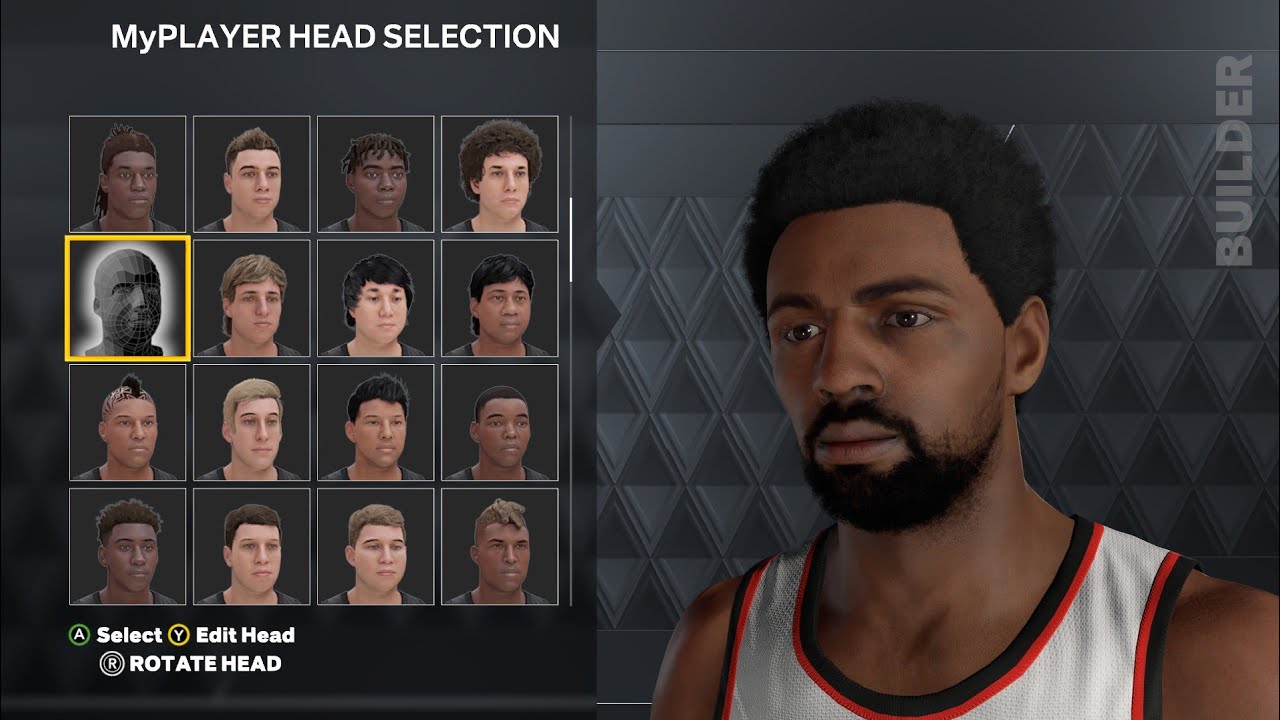This image appears to be a screenshot from a video game, likely an NBA basketball game on a console such as Nintendo, GameCube, or PlayStation. On the left side of the screen, there is a dark gray section displaying a grid of character faces organized in rows of four, essentially forming a 4x4 grid. These faces represent various basketball players, all male, and they come in different skin tones and hairstyles.

One specific character is highlighted with a yellow box, indicating it is currently selected. This selected face lacks distinguishable features, possibly implying the option to create a custom player. 

At the bottom of the screen, there are control prompts: "Press A to select," "Press Y to edit the head," and "Press R to rotate the head."

On the right side, more details are provided about the highlighted player. This character is a black man with a short black beard and short black hair. He is dressed in a white jersey with red and black trim, typical of a basketball uniform. The background behind him includes gray diamond shapes, and the word "Builder" is displayed vertically in the upper right-hand corner. 

Although the specific game is not mentioned, all elements suggest that this is a player selection or customization screen from an NBA-themed video game.